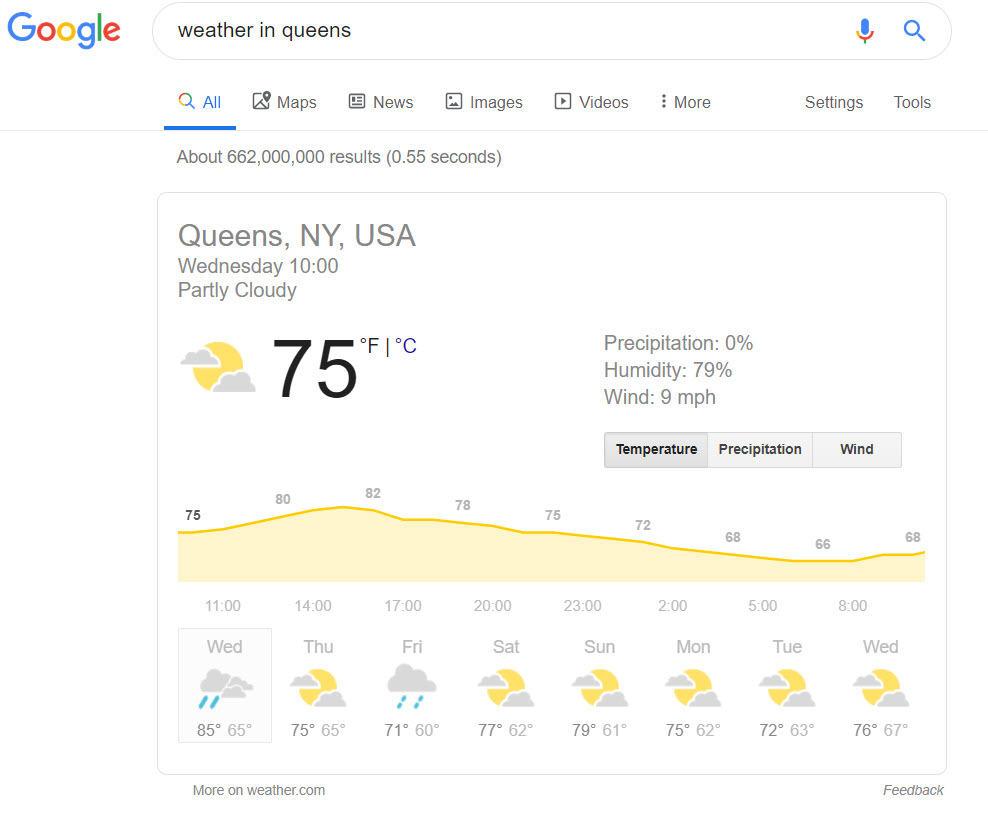A Google search result page for "weather in Queens" is displayed on the screen. At the top, the familiar Google logo in its colorful format is seen next to the search bar. Below the search bar are the navigation options: "All," "Maps," "News," "Images," "Videos," and "More," with "All" being highlighted. Additionally, options for "Settings" and "Tools" are accessible.

The search yields approximately 662 million results in 0.55 seconds. Dominating the center of the page is a white box with a gray outline that presents the current weather in Queens, New York. It specifies that it's Wednesday at 10 AM, with partly cloudy skies and a temperature of 75°F (with an option to switch to Celsius). An icon depicting the sun partially obscured by clouds is displayed.

The weather forecast details the hourly conditions from 11 AM to 8 PM, indicating no precipitation, 79% humidity, a wind speed of 9 mph, along with corresponding icons and metrics for temperature, precipitation, and wind.

Below this hourly chart, there is a seven-day weather forecast starting from the current Wednesday through to the next Wednesday. For each day, corresponding weather icons, high and low temperature predictions, and conditions are provided. The current day, Wednesday, is highlighted with a rain icon, showing a high of 85°F and a low of 65°F.

At the bottom of the weather box, there's a link labeled "More on weather.com" for additional details, with a "Feedback" option to its right. The entire content is set against a clean, white background.